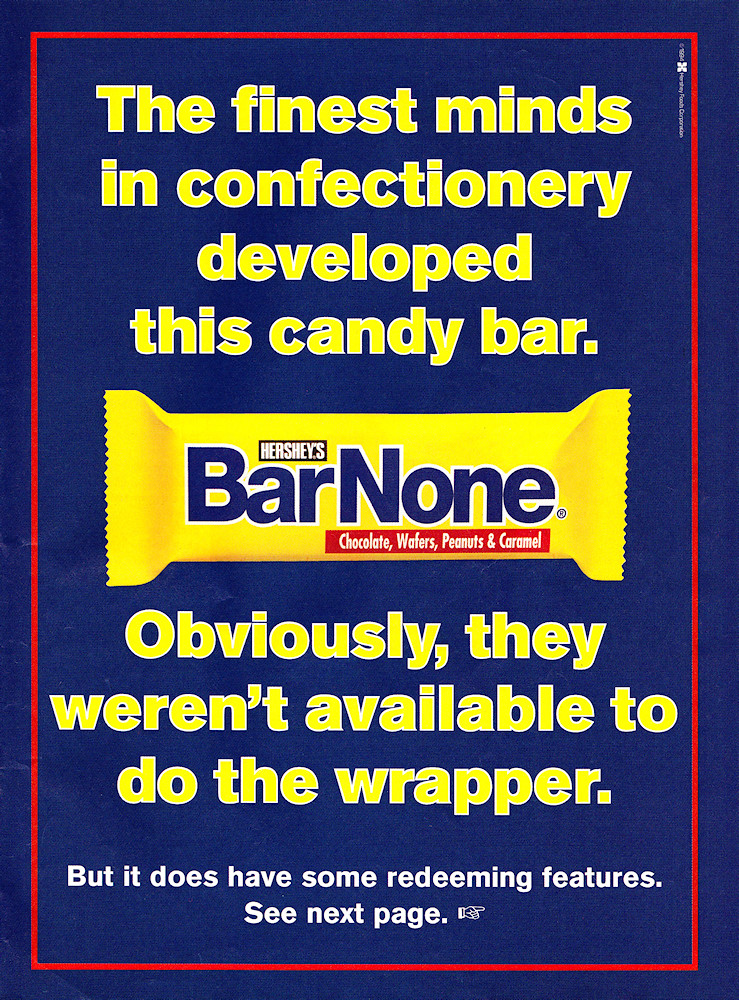The advertisement is a single-page poster with the dimensions suitable for a magazine. It features a dark blue background and is bordered by a thin red rectangular line. In the center of the poster, there is an image of a Hershey's "Bar None" candy bar in a yellow wrapper. Printed on the wrapper in blue font is "Bar None", and beneath that, in white font with an orange background, are the words "chocolate wafers, peanuts & caramel."

At the top of the poster, in yellow text, are the words: "The finest minds in confectionery developed this candy bar." Below the image of the candy bar, also in yellow text, it reads: "Obviously, they weren't available to do the wrapper." Following that, in white text, it says: "But it does have some redeeming features. See next page." Adjacent to this text is a small icon of a hand with a pointing finger, directing attention to the next page. There are also some additional words in white running along the top right side of the poster.